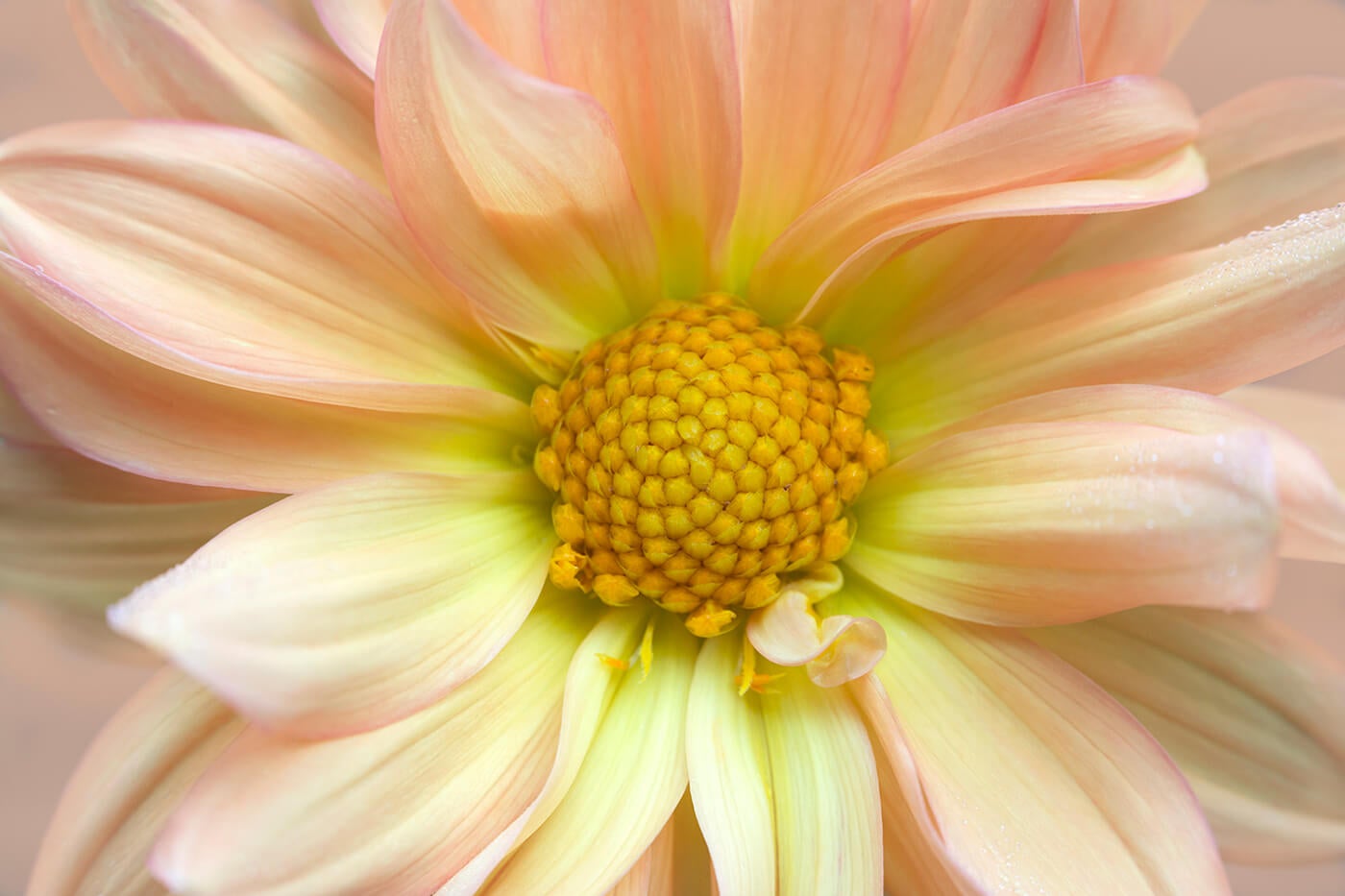This extreme close-up photograph captures the intricate details of a flower that resembles a daisy or chrysanthemum. The main subject is a fully open blossom with densely layered, medium-sized, oval leaf-shaped petals that are a very light pink hue, transitioning to a subtle green at their base. The edges of each petal have a delicate pink tint, creating an ethereal look. At the center of the flower is a vibrant yellow core, surrounded by a neon yellow glow which almost gives a greenish ring effect. The densely packed yellow pistil adds to the photo's intricate detail. The flower occupies the entire frame, showing about eight prominent petals but implying more in the background. This highly detailed image has no insects, animals, writing, people, buildings, or any other objects, drawing complete focus to the flower's delicate and mesmerizing features. The photograph's clarity makes it almost appear as a piece of photorealistic artwork.